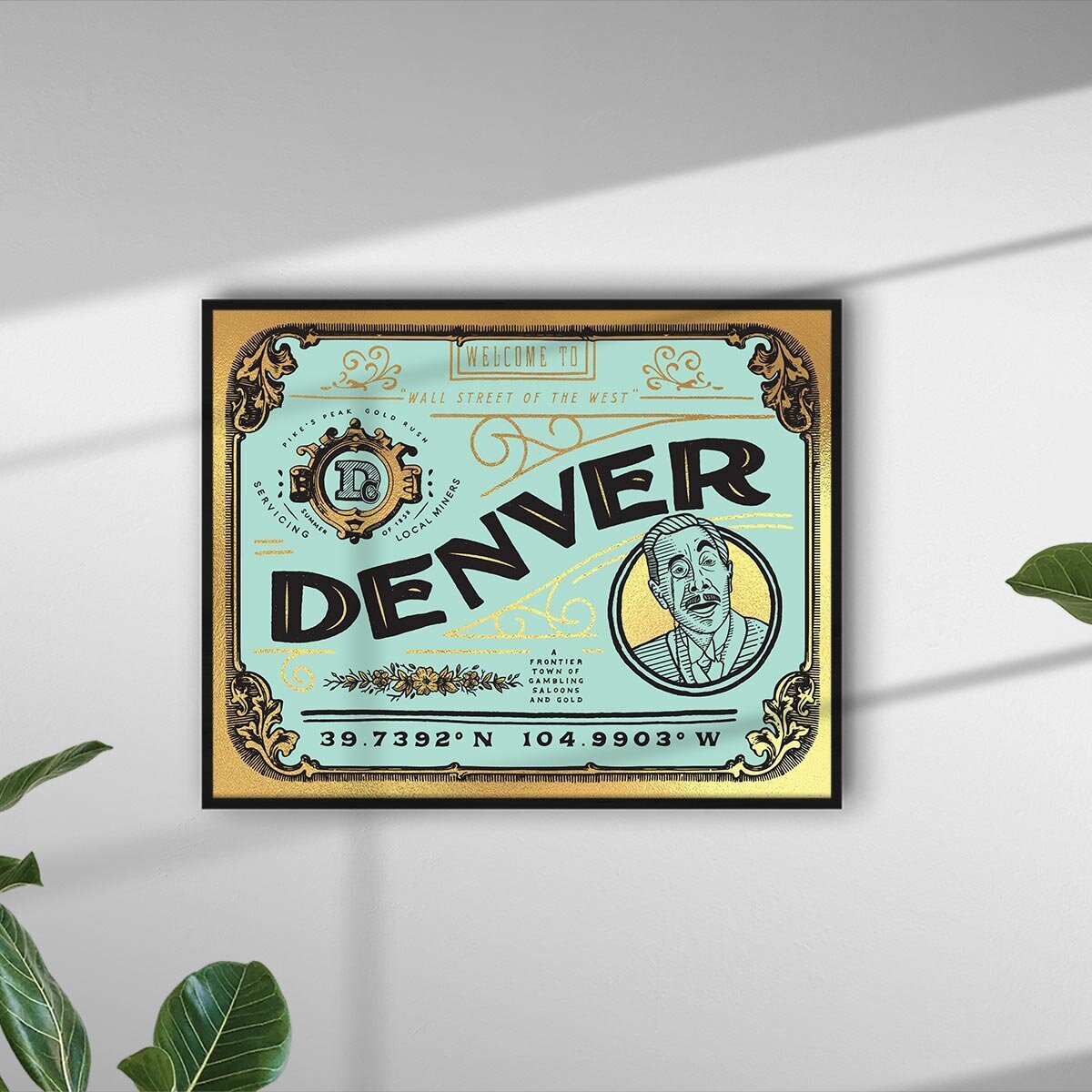The image showcases a detailed photograph of a rectangular framed poster mounted on a light gray wall. The frame is sleek and black, encasing a creatively designed poster. The poster features a light blue rectangle with rounded corners, bordered in gold. Dominating the center of the rectangle, the word "Denver" is presented in bold, black uppercase letters. 

Above this central element, in small gold font, is the welcoming phrase "Welcome to Wall Street of the West." Below "Denver," the coordinates "39.7392°N 104.9903°W" are displayed, pinpointing Denver's location. At the bottom right of the rectangle, there's a circular seal illustrating a long line drawing of a man with a monocle, neatly combed hair, and a suit. To the upper left corner, a coat of arms featuring a "D" symbol is present.

Surrounding the main elements and interspersed throughout the poster are intricate, decorative designs including floral motifs. The wall behind the frame, gray in color, captures shadows likely cast from window panes, adding a layer of texture to the background. In the lower left corner of the image and along the right edge, green leaves from indoor plants add a touch of natural color to the scene.